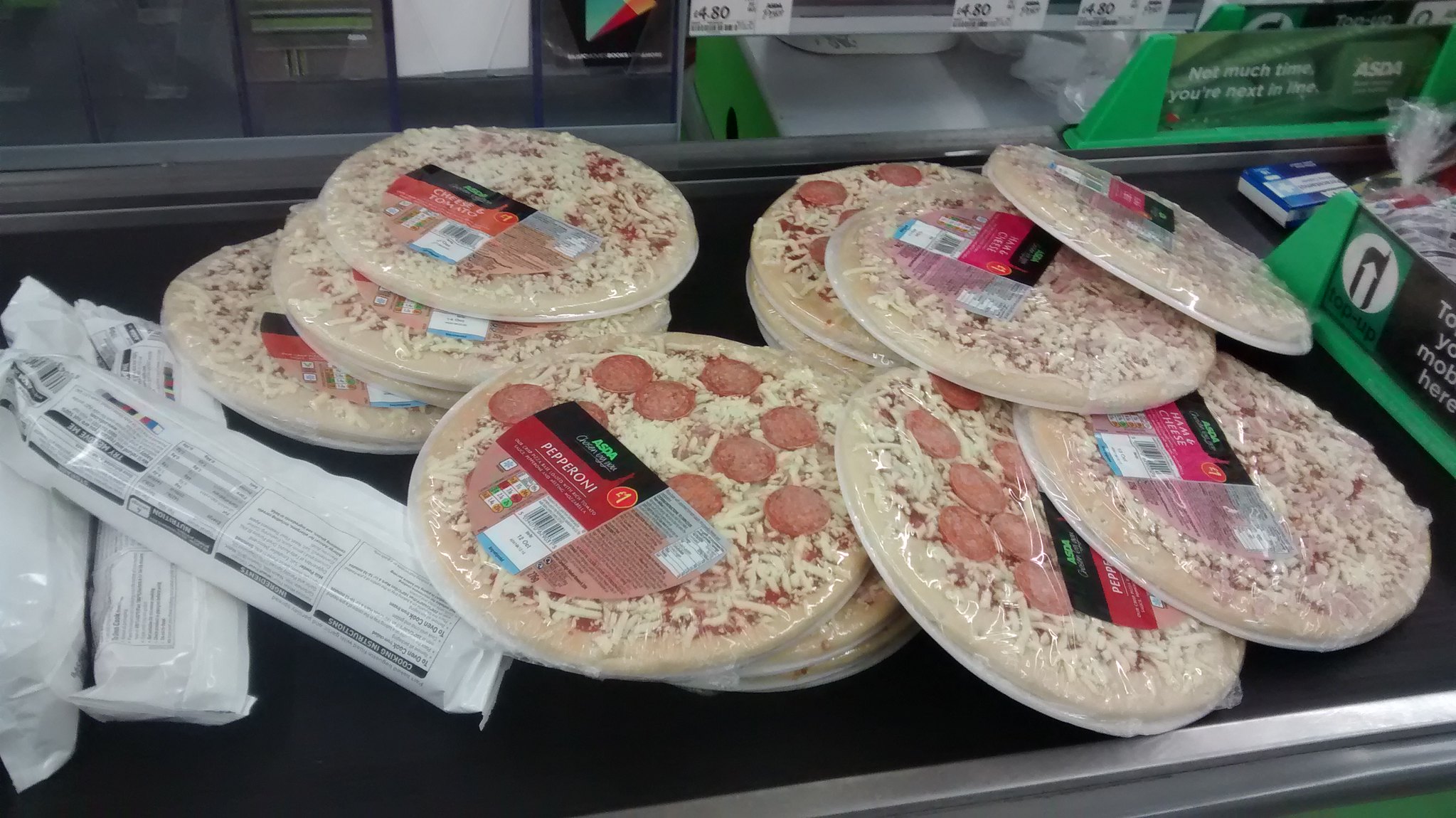This image captures a bustling moment at a grocery store checkout line, centering on a black conveyor belt flanked by metal sides. Dominating the scene are approximately 15 frozen pepperoni pizzas, neatly stacked in three piles, though one stack appears to be toppling over. These pizzas, encased in clear plastic wrap, reveal visible layers of cheese and pepperoni, with distinctive half-moon shaped stickers labeling them as pepperoni pizzas. Interspersed among them are a few other varieties, possibly tomato and ham and cheese, but their labels are less clear. 

On the left side of the conveyor belt, three rectangular packages wrapped in white plastic with some unreadable text lie in various orientations—two positioned vertically and one slightly angled. Speculations suggest they might be loaves of bread or rolled crusts, though the exact contents are obscured.

A green, white, and black divider is placed on the belt to separate this person's items from the next customer's groceries. In the background, partially visible price tags and store logos add to the everyday atmosphere. The overall setup encapsulates a familiar grocery shopping experience, highlighting the utilitarian nature of the conveyor belt in moving items towards the cashier.